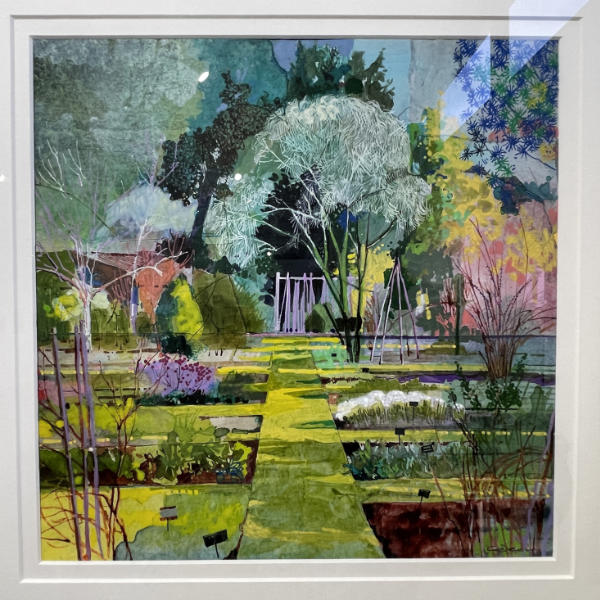This framed painting, likely from the late 19th or early 20th century, exquisitely captures a lush, vibrant garden scene with intricate details and a rich palette. The painting features a green, grassy path that winds through and around small rectangular lots, each showcasing different species of plants and vibrant flowers arranged in rows. The foreground is marked by a prominent leafless tree branch, adding depth to the scene. The background boasts a variety of trees, including what appears to be a willow and various other trees displaying striking autumnal hues. The garden is painted with a myriad of colors—bright pinks, crimson, white, blue, lavender, yellow, purple, and different shades of green, creating a vivid and dynamic visual experience. The green pathways crisscross horizontally and vertically, almost forming a maze-like pattern, enhancing the complexity and beauty of the setting. This remarkable work of art is a testament to the artist’s skill in blending diverse colors and elements to depict a visually stunning botanical garden.